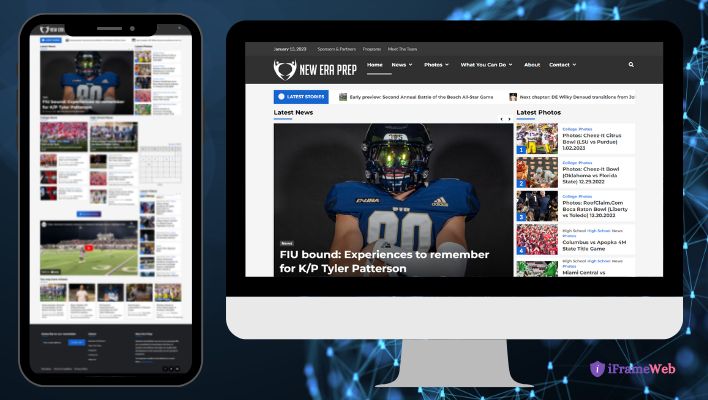The image is a collage featuring various elements. On the left side, the background transitions through different shades of blue, ranging from navy blue to lighter blue hues, interspersed with light blue lines. The bottom right corner of the image displays a purple shield with indistinct white markings, and nearby, the word "I" appears in purple, while "frame" is in pink.

Central to the collage are two screens: a black phone screen on the left and a desktop monitor on the right, both showing similar content. The desktop monitor features a mostly black display with a white section at the bottom. Despite the small size of the text on both screens, the content is consistent across devices, displaying the phrase "no error prep."

Above the screens, a navigation bar includes menu items in white text: Home, News, Photos, What You Can Do, About Us, and Contact, accompanied by a white magnifying glass icon for search functionality. Below the navigation, the heading "Latest News" appears in black, with "Latest" underlined.

Also part of the layout, a blue rectangle with a white circle and the word "latest" (partial view) is positioned above a photographic cutout of a football player. The athlete wears a blue and white jersey with an Adidas logo, a black helmet, and his arms are crossed, obscuring his jersey number.